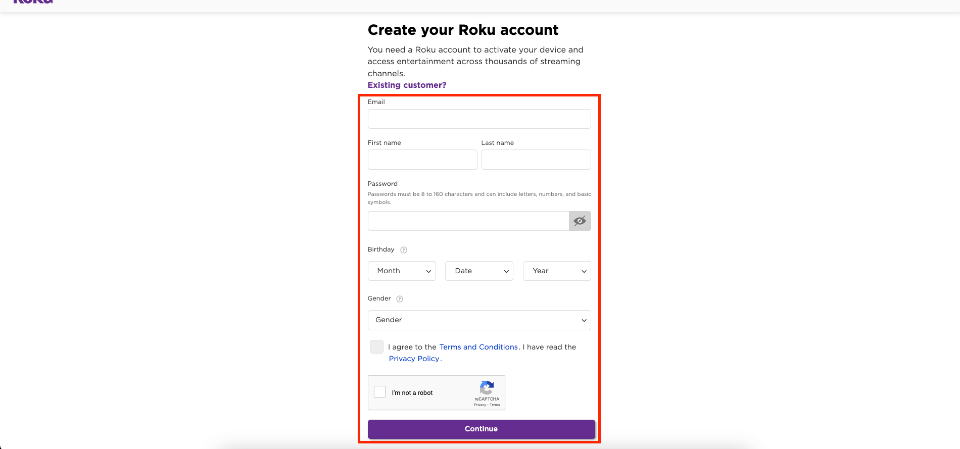This is a detailed screenshot of a user interface, either from a phone or a computer screen, showcasing the process of creating a Roku account. At the very top of the screen, in bold black letters, the text reads "Create your Roku account." Just below this heading, in smaller black lettering, there is a subtext that explains, "You need a Roku account to activate your device and access entertainment across thousands of streaming channels."

Beneath this informative text, prominently displayed in purple text, there is a question that reads, "Existing customer?" Immediately below this question, there is a red-bordered section which contains multiple entry fields for user information.

At the top of this red-bordered section is a text box bordered in light gray, labeled "Email," indicating where users should type in their email addresses. Underneath the email entry field, on the left-hand side, there's another label that reads "First name," followed by a corresponding light gray-bordered text box. Adjacent to this, on the right-hand side, is the "Last name" label with its own text box in a similar gray border.

Moving further down, the interface provides a section for creating a password. The label "Password" is displayed above an elongated light gray-bordered text box. Directly below this label, in very small black letters, is an important note detailing the password requirements: "Passwords between 8 to 180 characters and must contain letters, numbers, and symbols."

To the right of the password entry field, there's a smaller, darker gray-bordered box featuring an icon of an eyeball that is crossed out, typically indicating the option to toggle password visibility. This strikingly detailed interface is clearly designed to guide users through the necessary steps to establish their Roku account.